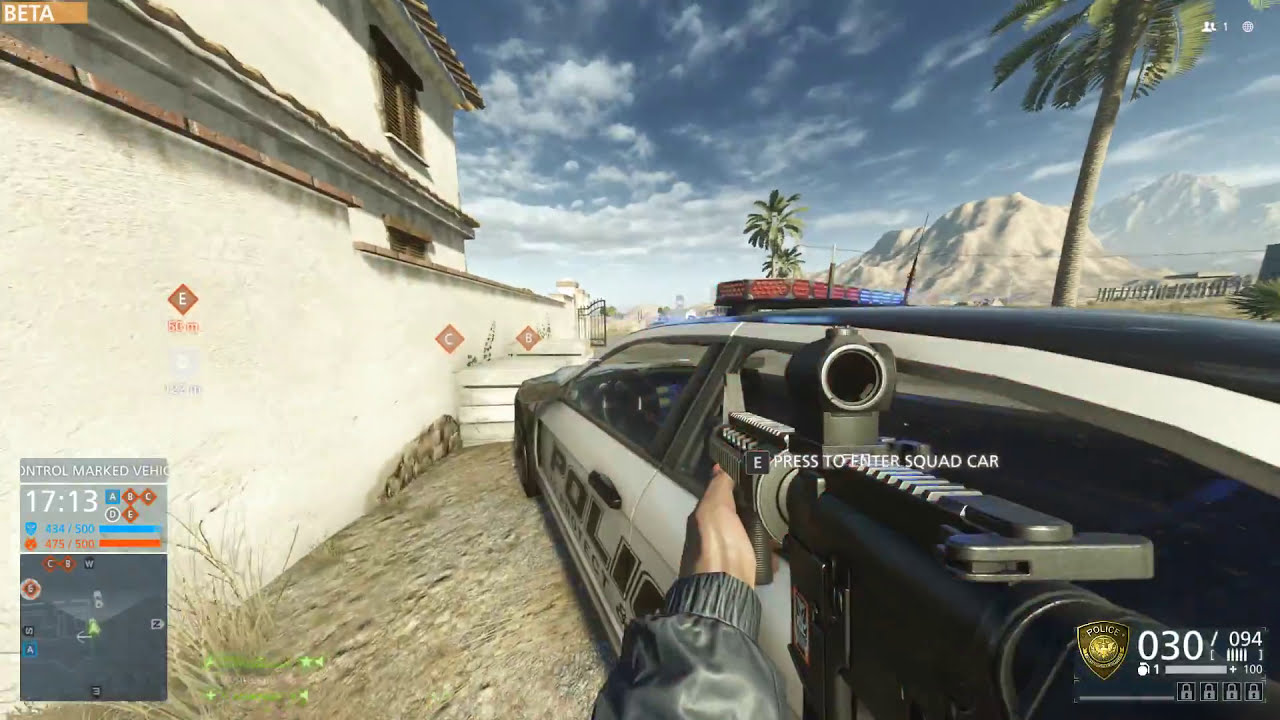The image is a detailed screenshot from a shooter video game, presenting the player's perspective. The player is holding a high-tech machine gun, supported by a hand in a grey jacket, pointing forward. Displayed at the top of the screen are the instructions "Press E to enter squad car," indicating interaction with a nearby black-and-white police car, specifically positioned at the back door on the driver's side. The setting features a sandy and gravelly ground next to a white stucco two-story building with visible steps and an upper window. A concrete wall within the scene displays the letters E, C, and B in diamond shapes. In the distant background, snow-capped mountains and a palm tree are visible under a blue sky with fluffy white clouds. The bottom left of the screen shows a control panel with text "30 / 095" and "Control marked vehicle 17:13," alongside a mini-map illustrating the player's position and surroundings.